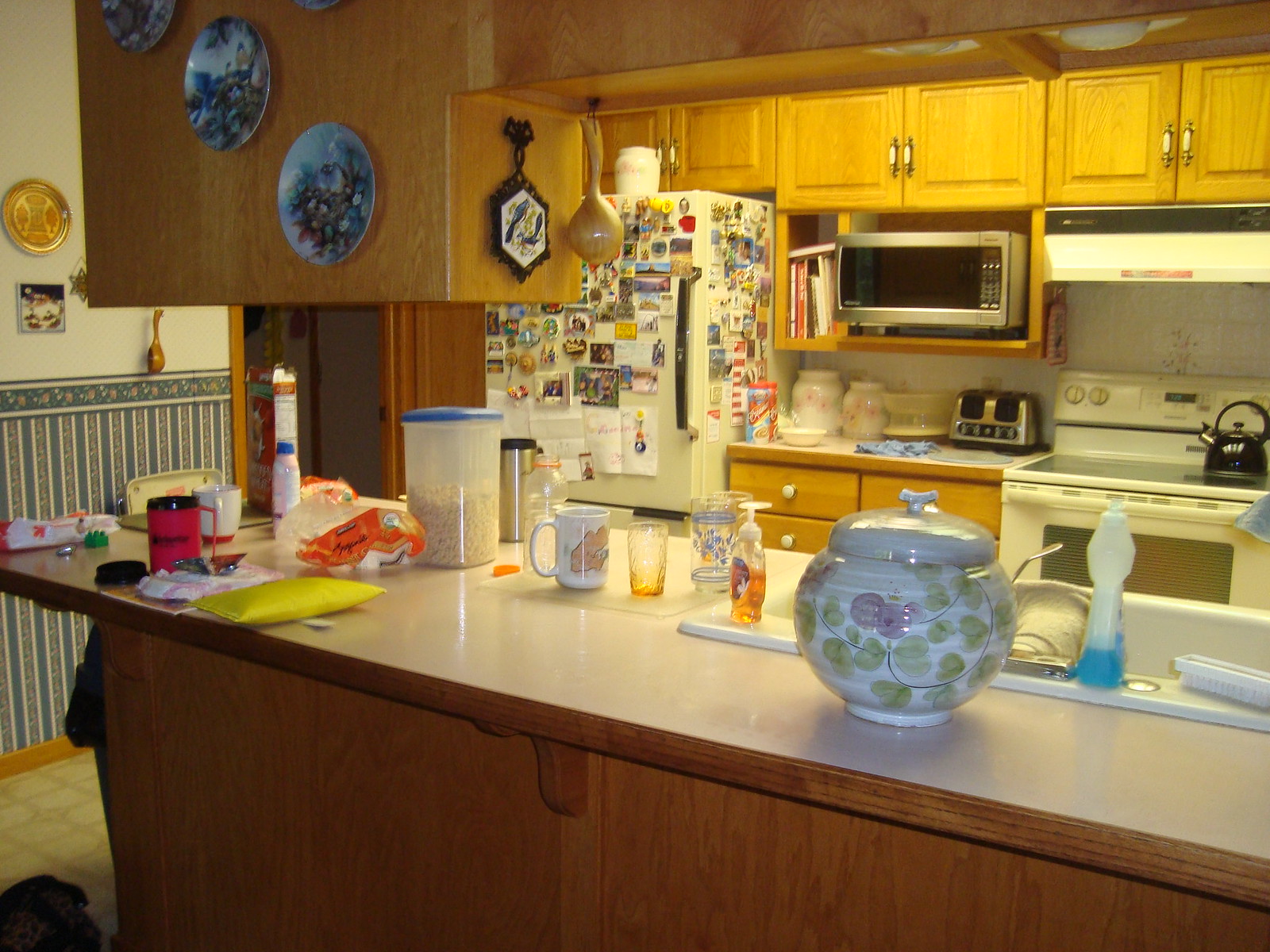The photograph captures the interior of a cozy kitchen centered around a white countertop, which forms an island with brown paneling underneath. Atop the countertop, there is a large, round China sugar bowl adorned with a delicate watercolor green pattern. Adjacent to it, part of a white sink basin is visible, accompanied by a bottle of dishwashing liquid in blue and hand soap in orange. Scattered around are various objects including a white mug, a glass, and several other cups. Notably, there is a white cylindrical container filled with brown Cheerios, capped with a blue lid. A loaf of bread in a yellow package, a red mug with a black rim, and a smaller white mug are also present. 

On the floor, there appears to be a purse or bag nearby. Overhead, brown cabinets are equipped with blue and white China plates, and what looks like a smooth gourd is attached to the cabinets. 

In the background, the kitchen is lined with numerous cabinets, a silver microwave, a white oven and stove with a black kettle on top, and a silver and black toaster. A white refrigerator stands out, covered with a variety of colorful magnets on the front and the side. Additionally, a collection of cookbooks is situated next to the microwave. The scene encapsulates a lived-in, functional kitchen space filled with everyday items.